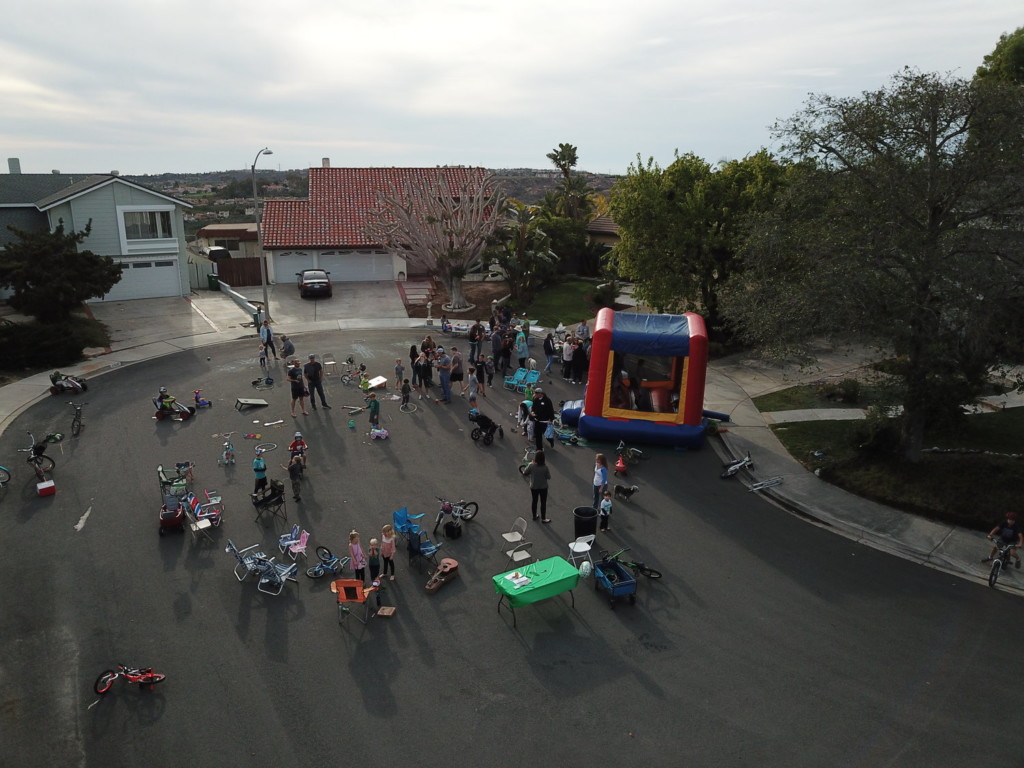This aerial drone photograph captures a lively scene in a residential cul-de-sac, nestled in what appears to be a semi-remote area. Centrally featured in the image is a children's party, with a square bounce house positioned just off the sidewalk on the right-hand side. Two houses are visible at the end of the cul-de-sac, with more residences faintly discernible in the distance. Approximately 30 children and 10 adults are gathered, creating a bustling atmosphere. The perimeter of the cul-de-sac is dotted with lawn chairs, tables, and assorted outdoor toys, including hula hoops, bicycles, scooters, and even miniature guitars. A prominent table with a green tablecloth stands at the front, surrounded by an array of colorful kid's bikes and scooters. The mid-afternoon sky is slightly overcast, setting a perfect backdrop for this cheerful community gathering.